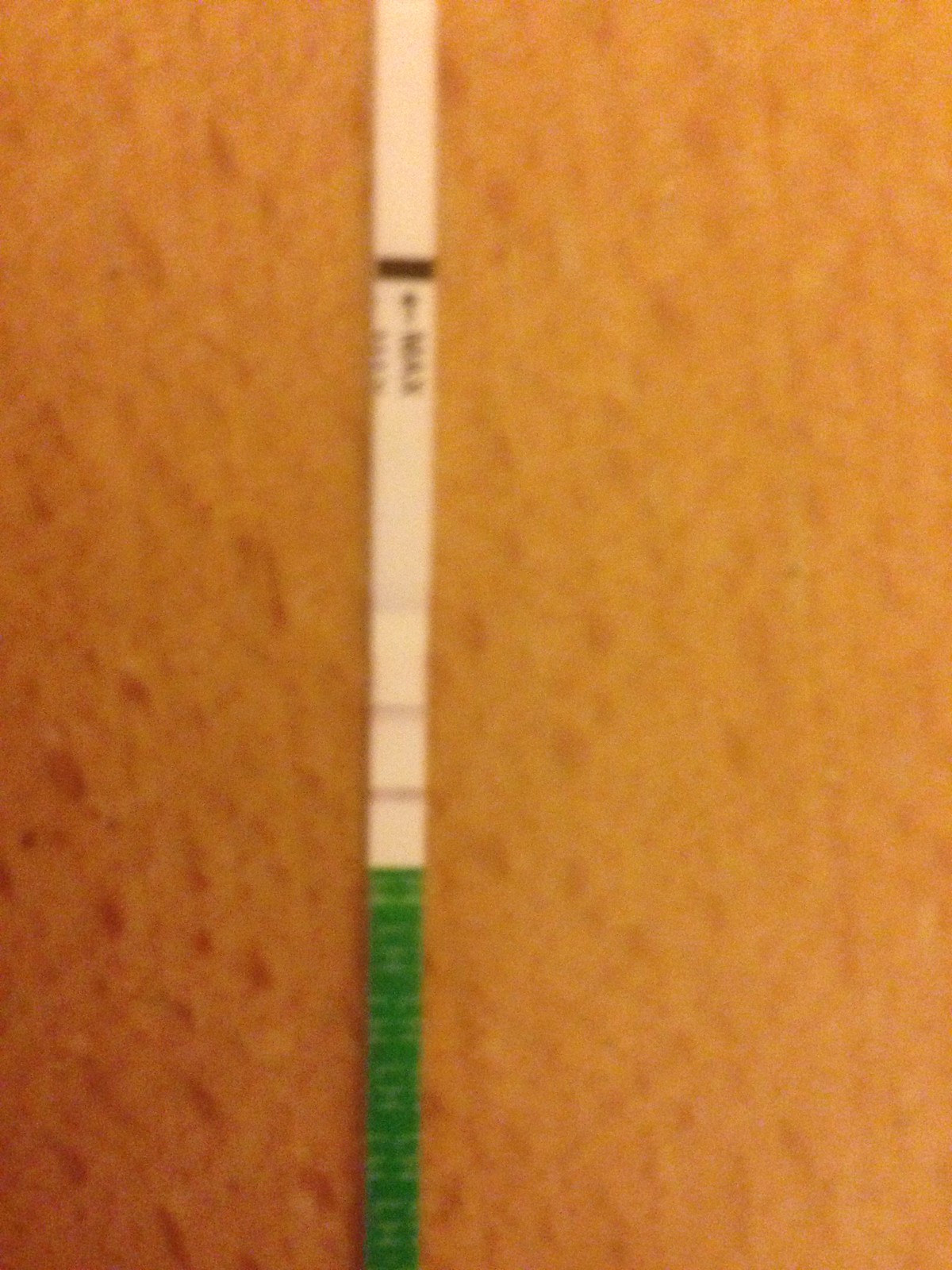The image depicts a close-up of a paper strip test, which could possibly be a COVID-19 or pregnancy test. The photograph is somewhat blurry, making details hard to distinguish. The test strip is placed vertically on an orange surface, likely a table. At the top of the strip, a black line runs horizontally, accompanied by an arrow and some indistinct lettering that appears to read "MAX." Midway down the strip, there are three red lines, with the top line appearing fainter than the two below it. The bottom third of the strip is tinged with a green color. The overall quality of the photo is low, with significant blur reducing clarity and making the identification of finer details challenging.